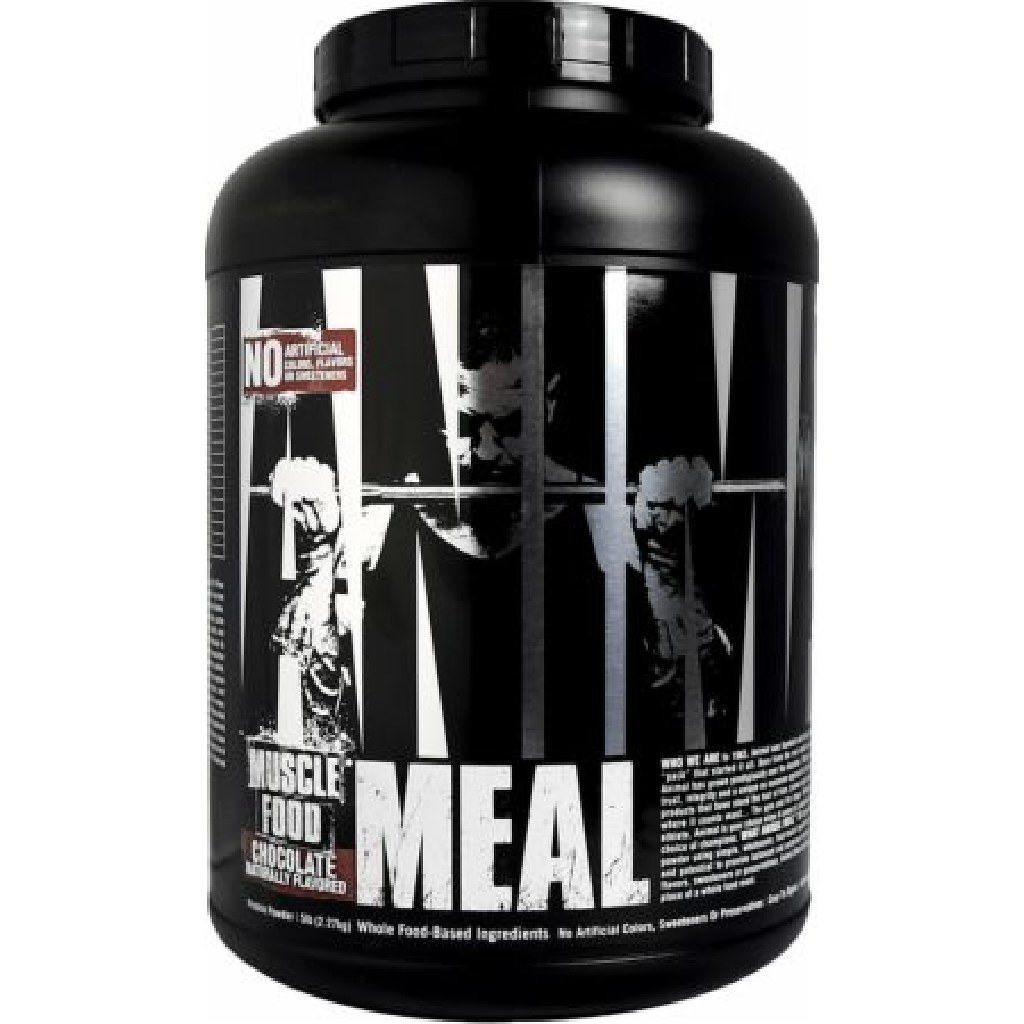The image features a large black plastic jug, akin to a gallon-sized container. The jug has a broad, screw-on black cap that spans approximately 80% of the container's width, making it easy to scoop out contents without touching the sides. On the front, there is a striking two-tone black and white image of a man lifting weights, who is wearing a dark tank top and has tattoos on his arms and hands. The man’s image is set against a possibly silver background, with white lines and elongated triangles accentuating the design.

Above the image, there is a sticker with a bold "NO" in white letters, indicating the absence of artificial colors, flavorings, and preservatives, although the text is partially obscured. Below the image, large white letters spell out "Muscle Food Chocolate Meal," suggesting this product is a dietary supplement or meal replacement targeted at weightlifters aiming to increase muscle size. Additional text along the bottom of the jug mentions "whole food-based ingredients," implying a focus on natural components. Despite much of the small print being illegible, the overall design is sleek and functional, clearly crafted for fitness enthusiasts. The jug is set against a clean, white background, enhancing its bold, black features.